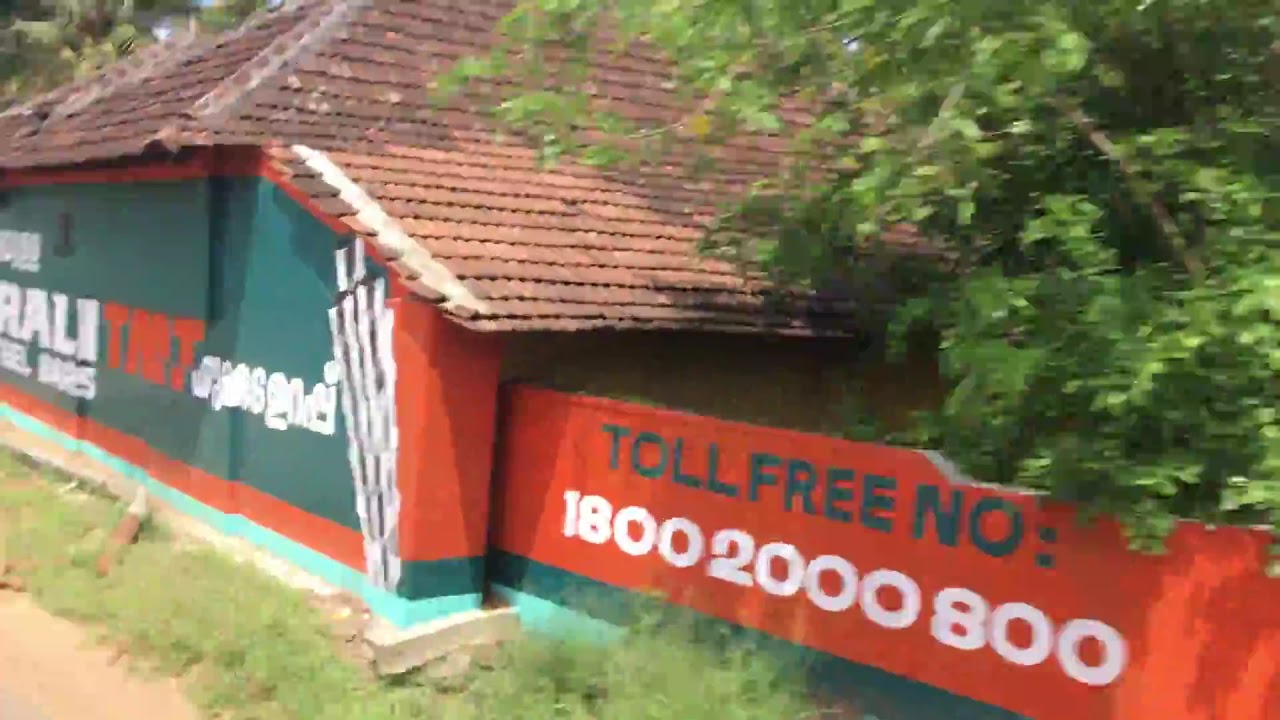The image depicts a somewhat weathered side of a house or business situated in either a South American or African country, viewed from an angle that includes a bit of fencing and surrounding greenery. The structure features a noticeable thatched roof made of burgundy bricks, which appears to need some maintenance. The wall of the building serves as a backdrop for a prominent sign that doubles as a part of the fence, painted in red with green stripes at the bottom. This sign, which could be made of wood or concrete, bears the toll-free number "1-800-2800" in white text, suggesting ease of contact. The left side of the image shows additional text on a larger wall, though it remains difficult to discern, and is in hues of blue and orange. The entire scene is set along a dirt road, with healthy green trees and some grass visible, adding a touch of nature to the somewhat rustic environment.